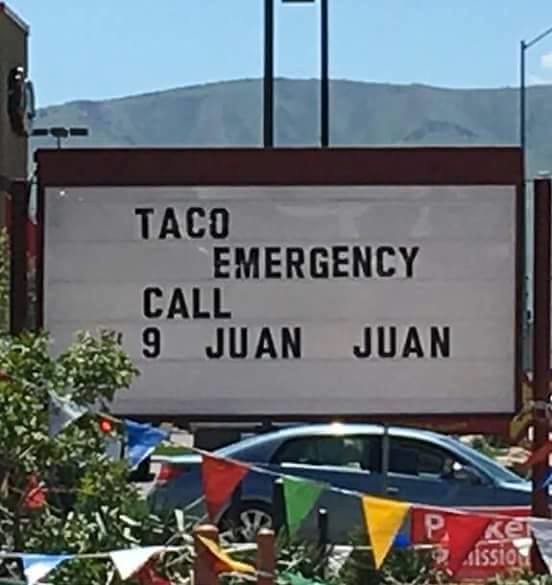The image captures a color photograph of an outdoor billboard-style sign situated on poles, likely outside a Mexican restaurant set against a picturesque mountainous backdrop under a clear blue sky. The sign, with a white background and black text, humorously reads, "Taco Emergency, call 911," playing on the pun "call 9-1-Juan." The sign comprises four lines of black letters, which are aligned in rows that can be slid into place. Below the sign hangs a string of triangular multicolored flags featuring hues such as white, blue, red, green, and yellow. Situated in what appears to be a parking lot near a street, the scene includes several cars, one of which is a blue sedan facing to the right. Additional elements include a building to the left and some foliage, giving further context to the outdoor, sunny setting.